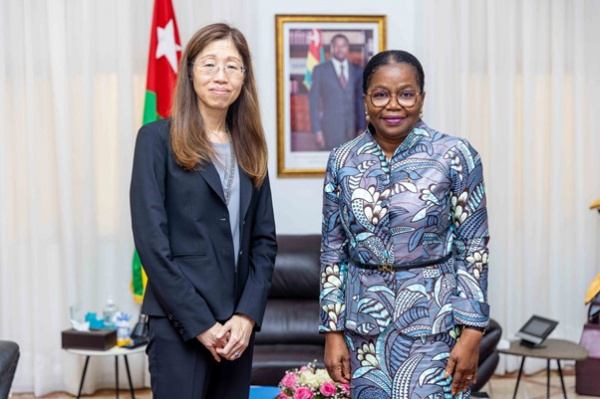In this detailed image, we see two women standing side by side. The woman on the left is Asian and has long, medium-brown hair. She is wearing glasses, a blue suit, and a matching blue shirt. To her right is a Black woman dressed in a blue patterned outfit with matching top and bottom. She also has her black hair pulled back and is wearing glasses. 

Behind them, there is a framed photograph of a Black man in a suit, prominently displayed on the wall. A portion of a dark leather loveseat or couch is visible below the photograph, as well as a floral bouquet featuring pink and white flowers. Flanking the couch are small end tables adorned with miscellaneous items, including what appears to be a tablet and a bottle of water. Additionally, a flag is partially visible behind the woman on the left, displaying the colors red, green, and yellow with a white star.